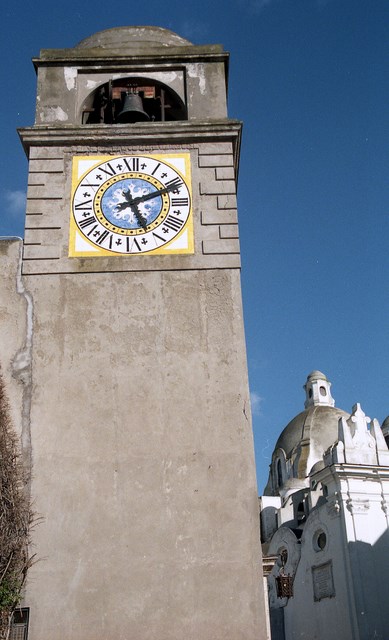This color photograph showcases a tall bell tower in a European town, likely from the late Renaissance period, made of gray concrete that appears somewhat discolored with white stains. The tower features a single black metal bell housed within an archway at the very top, with a small gray dome above it. Directly below the bell is a clock face within a yellow square outline. The clock, reading approximately 11 minutes past five, has black Roman numerals and hands on a white background, with a blue circle in the center adorned by a white snowflake-like design, all circumscribed by a yellow ring. The surrounding sky is mostly clear with a couple of minor clouds. To the right, in the background, stands a white domed building with cross-like ornamentation and smaller dome-topped cupola. Additionally, small white circles are present along the top of its walls, under one of which is a sign. A tree partially rounds the buildings, adding a touch of nature to the scene.